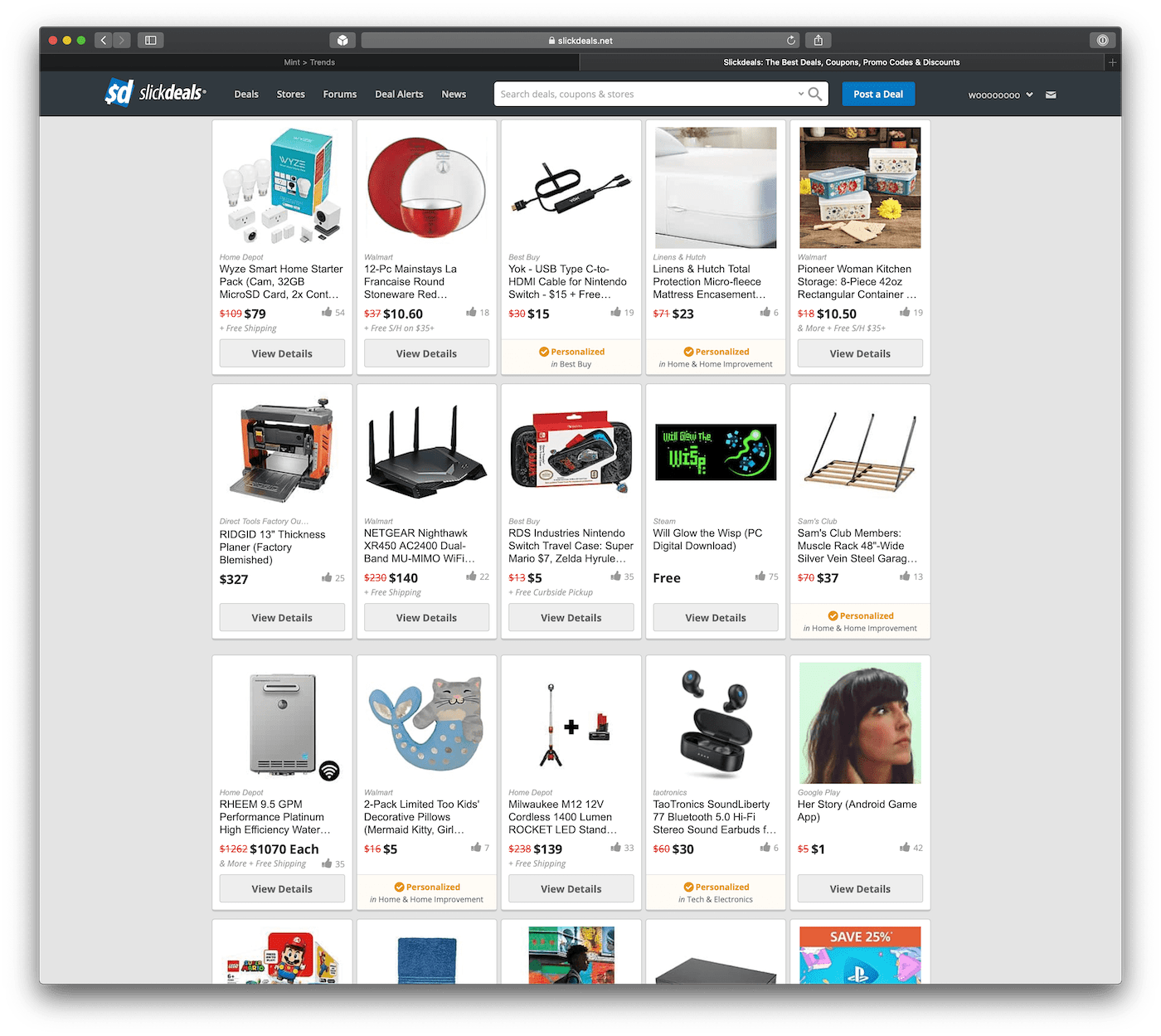This is a detailed screenshot of a Safari browser displaying the Sleek Deals website, characterized by a black header. The Sleek Deals logo, represented by the initials "SD" on a blue background, is prominently placed on the header's left side. Adjacent to the logo, the top navigation menu includes tabs labeled "Deals," "Stores," "Forums," "Deal Alerts," and "News." On the far right of the header, you'll find a search bar and a blue "Post a Deal" button.

The main section of the screenshot showcases a product listings page, divided into approximately 20 sections, each enclosed in white boxes. The first product featured is the "Waze Smart Home Starter Pack," which includes smart light bulbs. Originally priced at $109, it is currently on sale for $79. A "View Details" button is located at the bottom of this product box. 

The second product is a set of "12 Mainstays Stemware and Plates," initially priced at $37 and now discounted to $10.60. This product box also has a "View Details" button. This trend continues with most product listings on this page, offering a detailed view option. However, some items feature a different button labeled "Personalized In-Home and Home Improvement" instead.